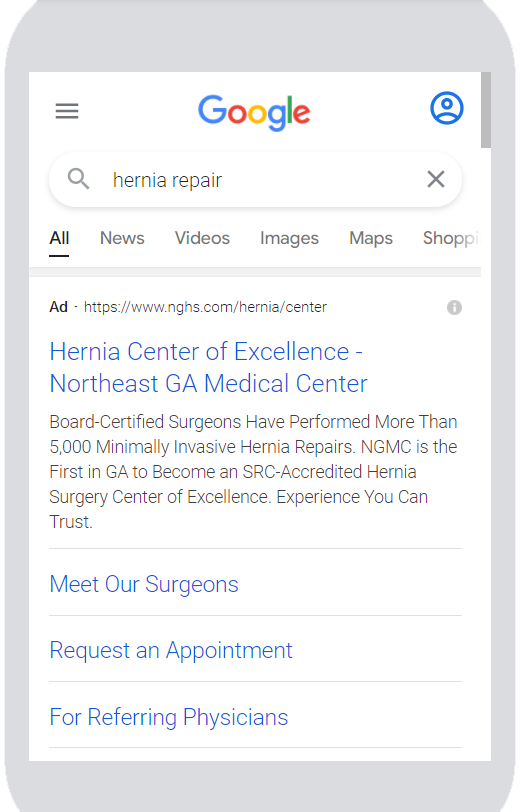The image is a screenshot of a Google search results page. At the top, the Google logo with its colorful design is displayed alongside a circular user icon. The central focus of the image is the search bar, which contains the text "hernia repair." To the left of the search bar is a magnifying glass icon, and to the right is an 'X' icon for canceling the search query. Beneath the search bar, there is a horizontal menu with various filter options including "All," "News," "Video," "Images," "Maps," and "Shopping," with "All" being selected.

Further down, the screenshot highlights a Google advertisement. The ad is marked with "Ad" in the upper left corner, followed by a URL and a small information button that offers more details about the ad. The title of the ad, in blue text, reads "Hernia Center of Excellence Northeast Georgia Medical Center." Below the title, there is body text associated with the ad, providing additional information about the center. There are also additional links underneath the ad's text, including "Meet Our Surgeons," "Request an Appointment," and "For Referring Physicians," which are presented as list items.

Overall, the screenshot serves as an illustrative example of how advertisements appear on a Google search results page, shedding light on the structure and elements of a typical Google ad.